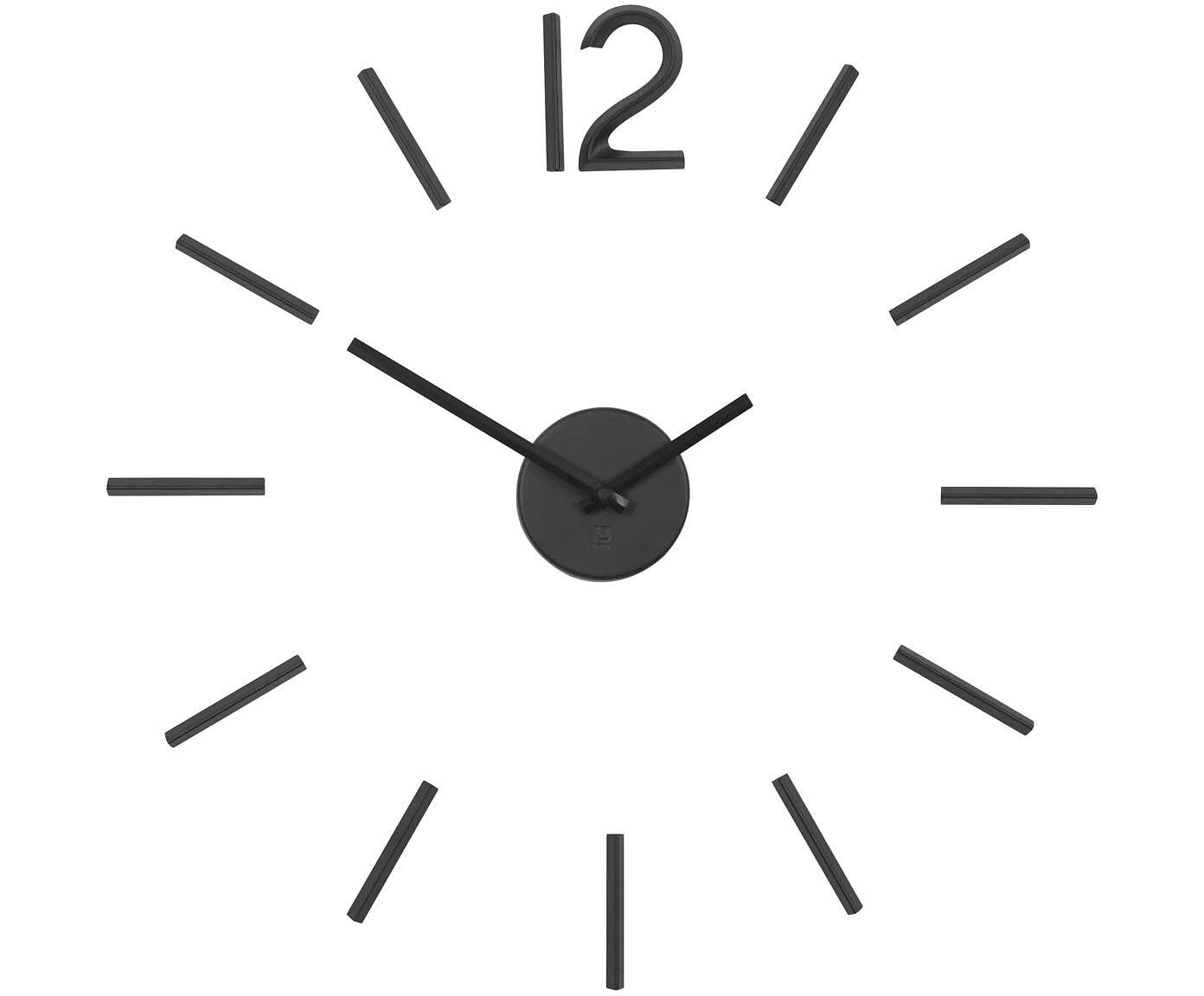This image is a minimalist computer rendering of a clock face set against a pure white background. The clock does not have any border or frame, and no shadowing is present. At the top, the number "12" is distinctly marked, while the rest of the hour positions are indicated by thin black lines of equal width, simplifying the design. The clock hands, also thin black lines matching the width of the hour markers, are positioned to show 10 minutes before 2. In the center of the clock, there is a small black metal circle from which the hands extend. The overall appearance is very simplistic, making it challenging to distinguish whether it is a digital graphic or an actual photograph.